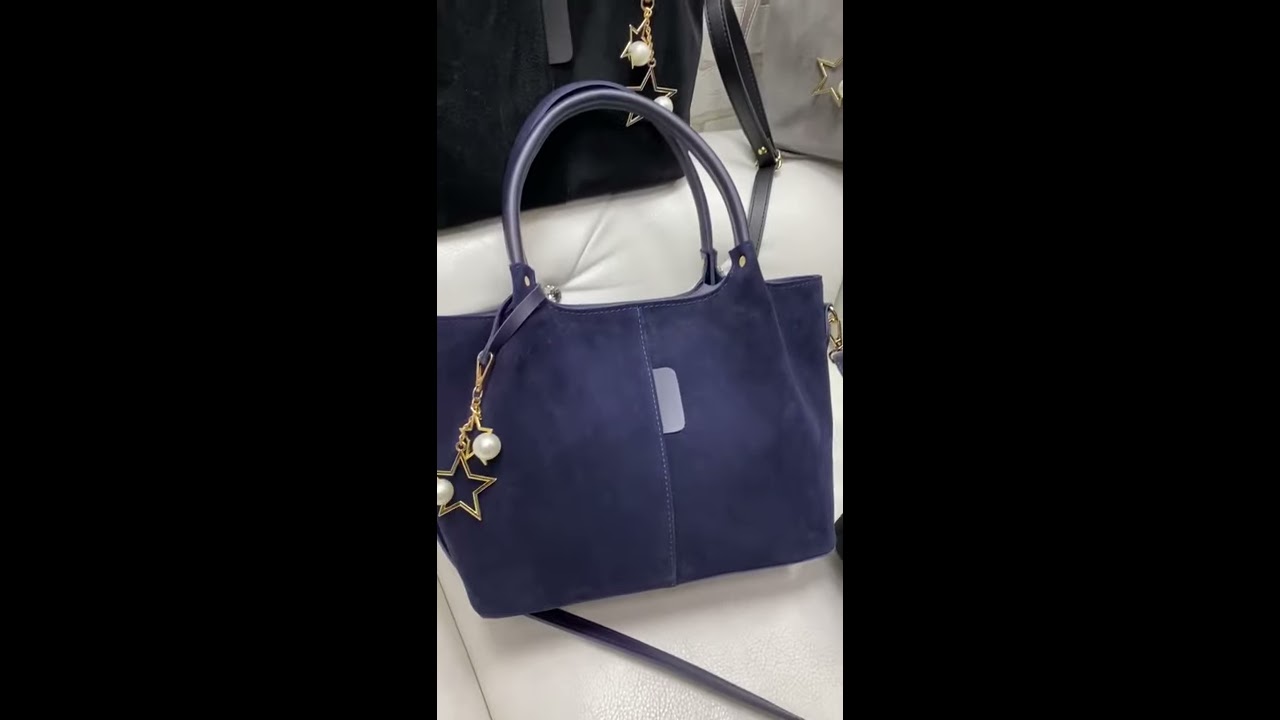The image captures an indoor setting, likely in a home, and appears to be a screenshot of a portrait-style photograph displayed on a phone screen, currently oriented in landscape mode. The central focus is a blue suede satchel-style purse with two handles, resting on a white leather surface, possibly a couch or armchair. The purse features a prominent gray label in the middle and a gold chain with decorative items, including two pearls and a star-shaped charm, hanging from one of its handles. In the background, there is a black purse with a similar decorative chain, positioned on what seems to be the raised arm of the same white leather furniture. The photograph is framed by black panels on both the left and right sides, suggesting it might be the center image of a triptych. Additionally, a small portion of another handbag, also adorned with a star charm, is visible in the upper right corner. The white surface beneath the purse shows an upholstered button, indicating it is part of a piece of furniture.